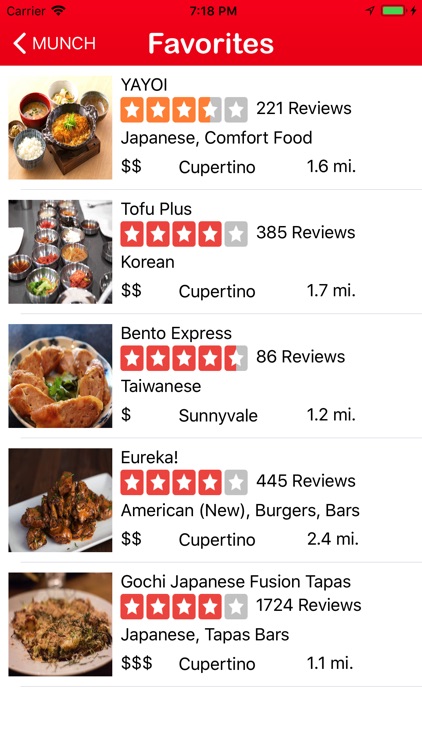Screenshot of a smartphone displaying a restaurant app. At the top, a horizontal red banner reads "Carrier" in black on the left, with a Wi-Fi icon beside it. Centered in the banner, the time reads "7:18 PM" in black, while the far right indicates that the sound is turned off. The battery icon is fully green, with a black lightning bolt indicating charging.

Beneath the red banner, the text "Favorites" appears in large white letters. To the left, in lighter white letters, "Munch" is displayed alongside a left-facing arrow.

The main section lists five restaurants with their details and images:

1. **Yayoi**
   - Rating: 3.5 stars out of 221 reviews
   - Cuisine: Japanese comfort food
   - Location: Cupertino, 1.6 miles away
   - Image: Traditional Asian dishes, bowls of rice

2. **Tofu Plus**
   - Rating: 4 stars out of 385 reviews
   - Cuisine: Korean
   - Location: Cupertino, 1.7 miles away
   - Image: A table with stainless steel bowls, each containing different items

3. **Bento Express**
   - Rating: 4.5 stars out of 86 reviews
   - Cuisine: Taiwanese
   - Location: Sunnyvale, 1.2 miles away
   - Image: A plate with crispy, fried items

4. **Eureka**
   - Rating: 4 stars out of 445 reviews
   - Cuisine: American (new burgers and bars)
   - Location: Cupertino, 2.4 miles away
   - Image: A pile of meatballs on a white plate

5. **Gochi Japanese Fusion Tapas**
   - Rating: 4 stars out of 1,724 reviews
   - Cuisine: Japanese tapas bars
   - Location: Cupertino, 1.1 miles away
   - Image: A white plate with stir-fry

All star ratings are white, displayed on orange square backgrounds.